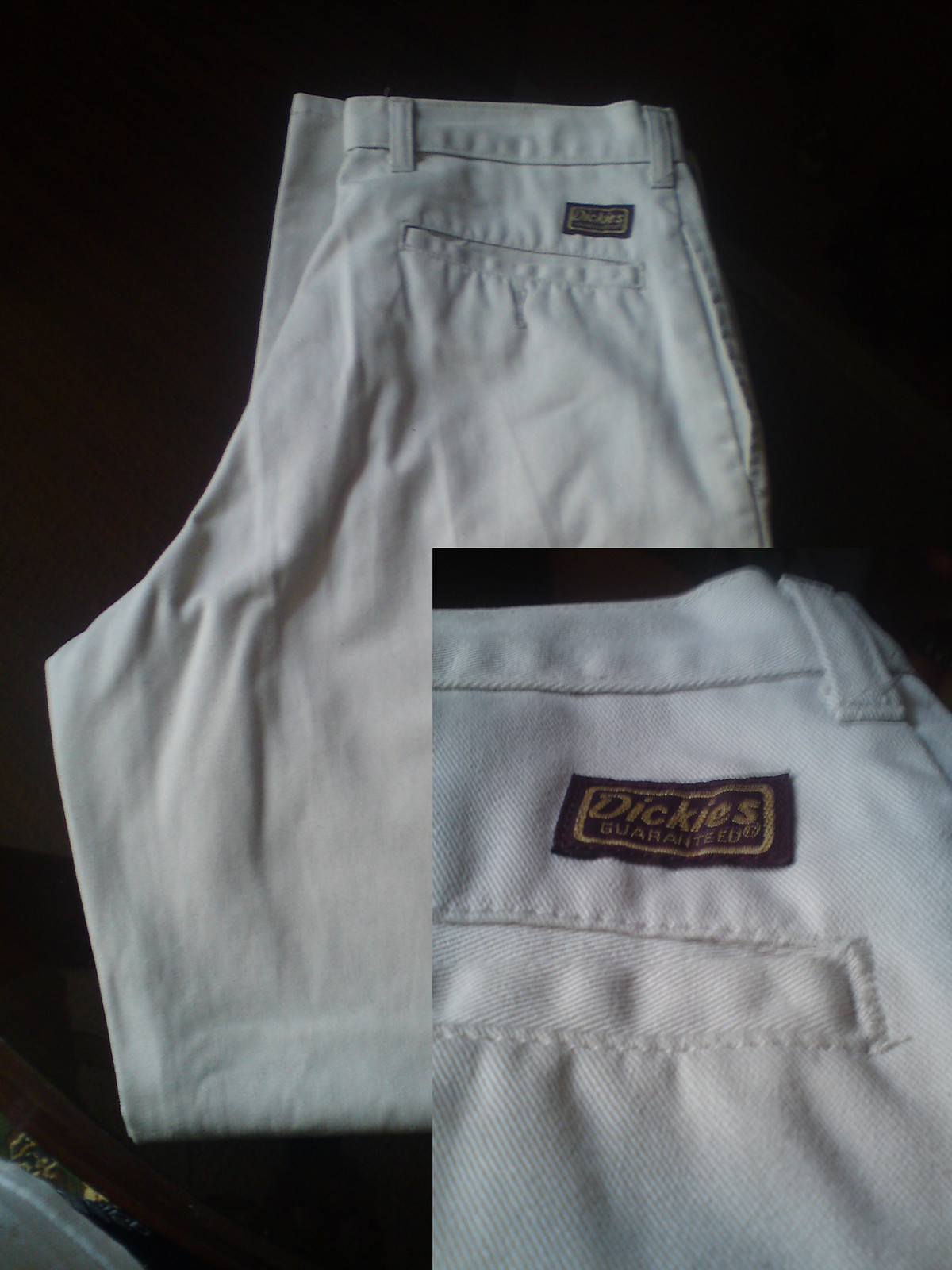The image features a pair of white Dickies pants, folded in half and positioned on a dark or black surface that could resemble the inside of a suitcase, given the presence of what appear to be gold letters or buckles. The pants, made of a heavy fabric typical of workwear, include belt loops and a back pocket. Positioned above the back pocket is a distinctive Dickies label with a black background and gold elements— the word 'Dickies' and 'Guaranteed' surrounded by a gold border. To the bottom right of the main image, there is a magnified inset showcasing the same pants’ back pocket area, prominently highlighting the Dickies logo and details of the tag for better visibility. Additionally, another white item of clothing seems to be partially visible in the bottom left corner of the photo.